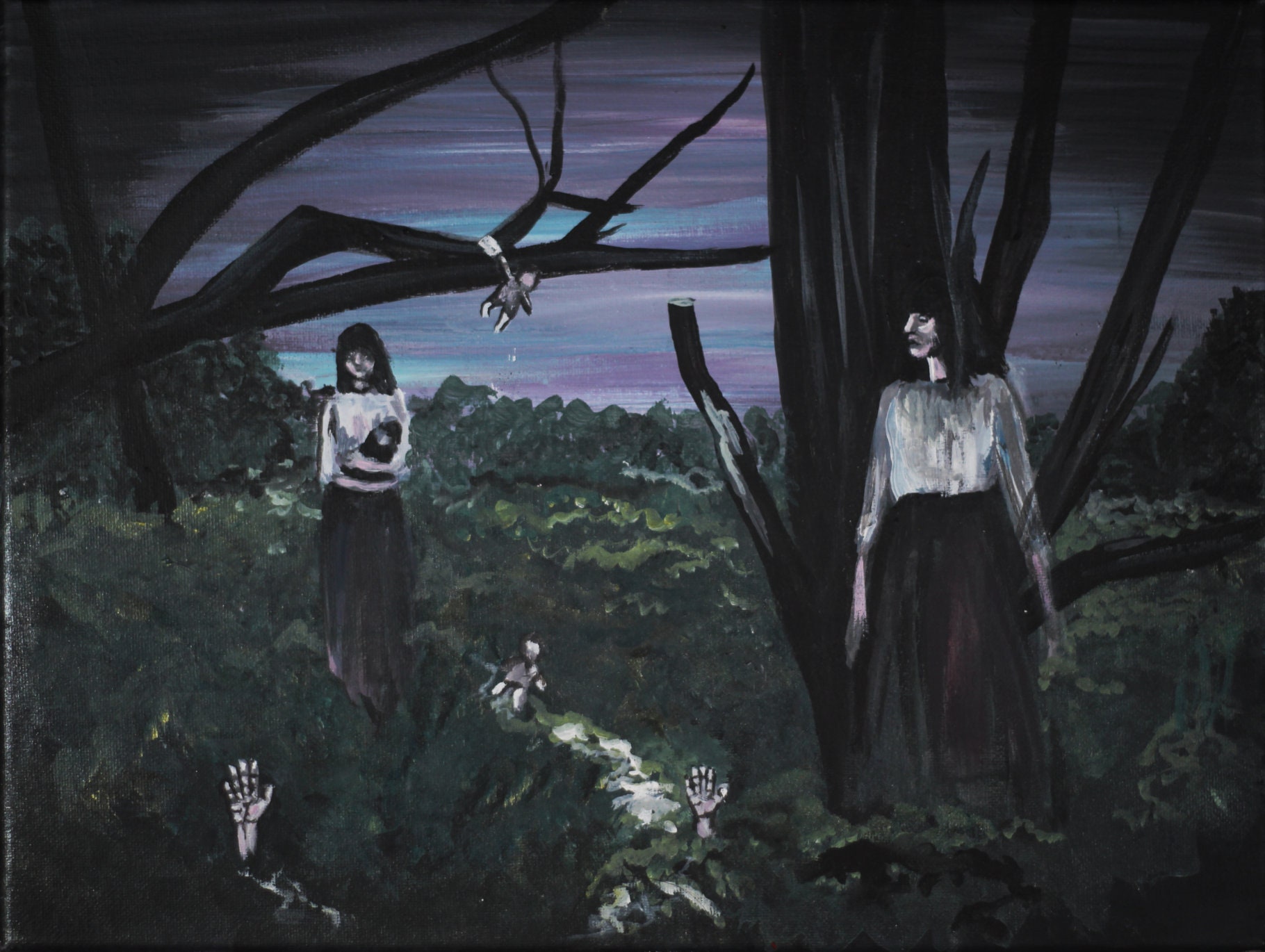The image is a dark, eerie painting, likely done in acrylics, depicting an outdoor nighttime scene. The sky transitions from a mix of purple and blue into a deep darkness. The setting appears to be a forest or an open field with tall grass and dark tree trunks stretching upward in the background. Central to the composition are two women with long black hair, white faces, and white tops paired with black skirts that reach down to their ankles. The woman on the right stands in front of a tree trunk with her head turned to the left, as if trying to hide behind it, her hands by her side. Further into the scene, the second woman, similarly dressed, appears to be holding a dark object that could resemble a baby carrier. The painting also features unsettling elements: hands eerily emerging from the greenish ground, and dolls—one lying on the ground and another hanging from a branch. The overall atmosphere is haunting and mysterious.